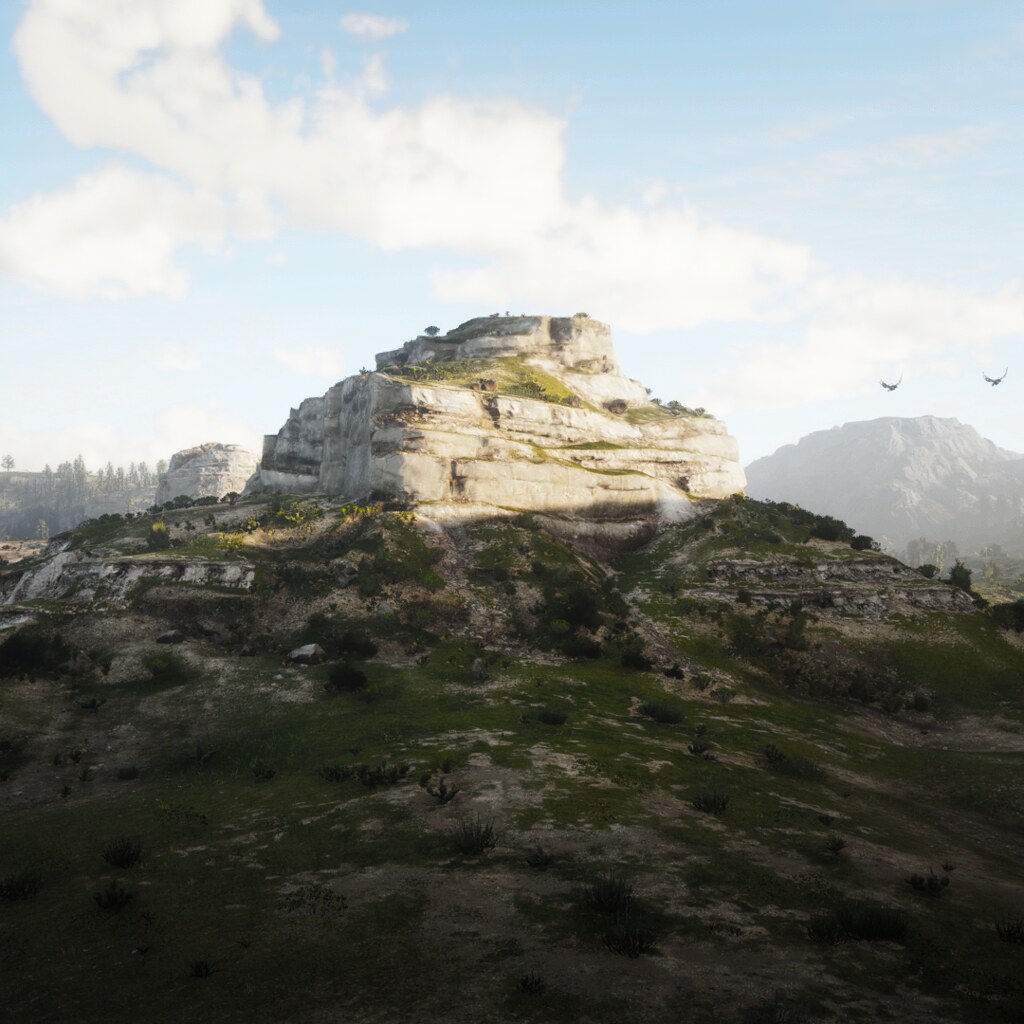This square image, likely a 3D computer-generated scene, depicts a picturesque mountainous region. Dominating the foreground is a gradually inclining hill characterized by a mix of green grass and patches of brown dirt. Atop this hill sits a prominent stack of white rocks with sparse green foliage, resembling another small hill or pyramid. This formation, almost square in shape, has small, scattered trees and bushes adorning its slopes. In the distance, another white mound is visible, partially veiled by mist, while further off to the right, a distant brown mountain fades into the horizon. The sky above is a serene light blue, dotted with semi-transparent, slightly white clouds. Adding to the dynamic atmosphere, a couple of birds are seen soaring on the right side of the image, their distinct shapes enhancing the scene's computer-generated quality.